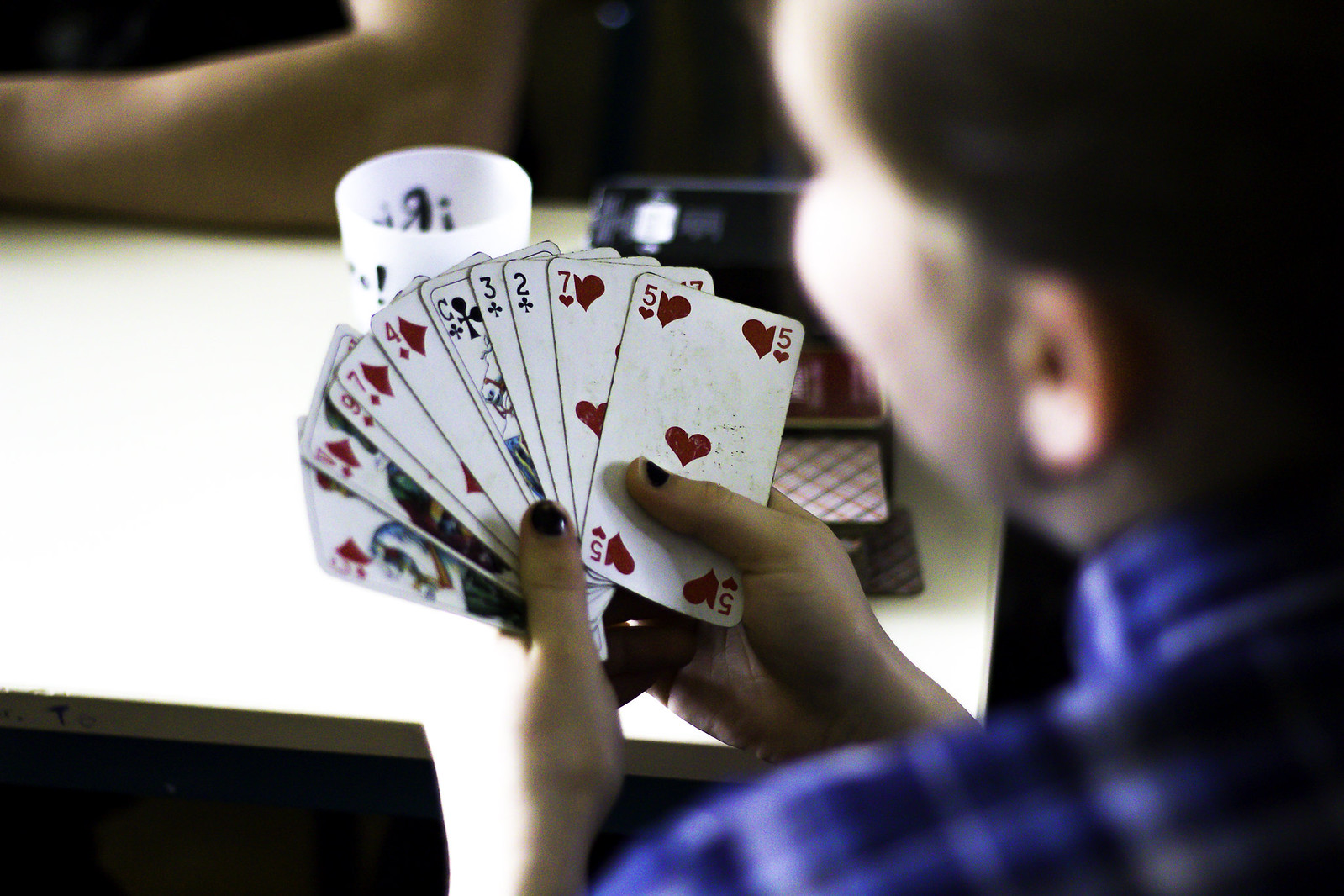The photograph captures a person seated at a table from an over-the-shoulder perspective, with the camera positioned above their left shoulder. The individual, whose upper body is mostly out of focus, is identifiable by a blue and white checkered collared shirt and brown hair that is either short or pulled back. They appear to be white, with visible Caucasian hands adorned with chipped black nail polish. The person's hands are holding a fan of playing cards, displaying at least eight or nine cards including the five of hearts, seven of hearts, and two and three of clubs. The rest of the cards are difficult to discern due to the focus. In the background, a white table is visible, featuring another stack of face-down playing cards and a white cup with black writing on it.